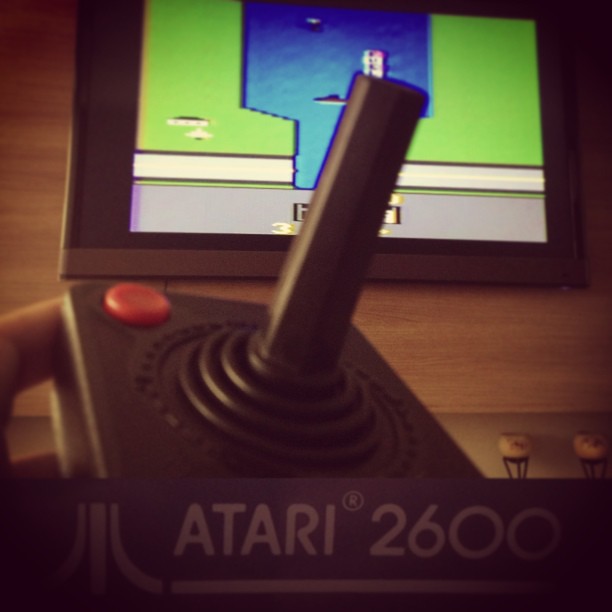An advertisement for the Atari 2600 is prominently displayed. The focal point is a black joystick, characterized by a black square base and a striking red button positioned at the top left corner. Surrounding the joystick are concentric rings leading up to the stick itself. The background features a wooden texture with visible grain patterns adding a rustic ambiance. At the top of the image, there's a screen displaying a retro pixelated video game. The game interface shows a black background with a gray bar running across the bottom. Within the game, green blocks appear on both the left and right sides, and a white stripe stretches horizontally across the scene, resembling a road. The lower part of the screen showcases a segment labeled with the number three in yellow, situated above a gray area. Additionally, the game appears to depict a body of blue water populated with indiscernible objects, enhancing the vintage gaming aesthetic.